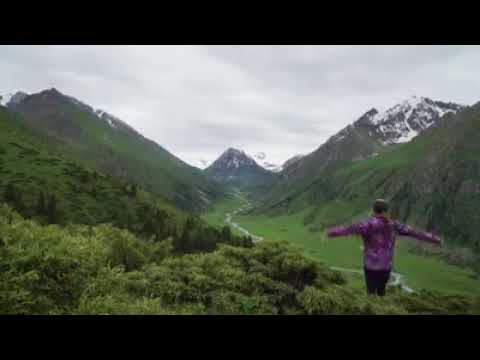In this image, a person stands prominently in the bottom right corner, posing with arms outstretched, resembling a T or airplane stance. The individual, outfitted in a dark pink shirt with lighter pink spots and black pants, appears to be positioned atop a tree, suggesting either a computer-generated context or a creative photo angle. The foreground features a sprawling field of bushes and trees in various shades of green. Beyond this, a river snakes through a vast valley, past a series of mountains. The mountains in the background are partially snow-capped, evoking similarities to the Alps, and include one triangular peak in the center and two smaller peaks to the right. The sky overhead is uniformly gray and filled with clouds, while horizontal black bars frame the top and bottom of the image, which seems horizontally stretched, indicative of a low-resolution or pixelated still from a video.